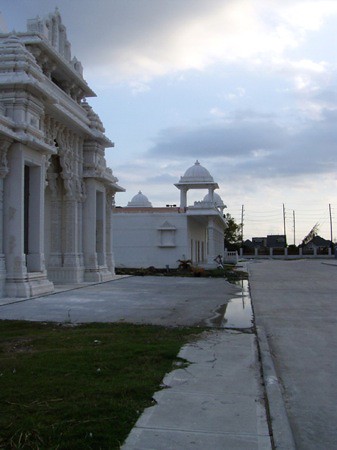The image captures a cloudy daytime scene where the sun is obscured, casting a bright glow behind dark-hued clouds. Dominating the left side are detailed white architectural buildings, likely inspired by Roman or Greek design, featuring domed caps set upon white pillars. At least two buildings are prominently visible, with hints of another structure discernible in the distance. The buildings have multiple roof levels and entrances on either side, with a ripple design. A concrete street and sidewalk, adorned with patches of green grass and puddles, stretch in front of these buildings. In the distance, telephone poles with wires, as well as what appear to be more dark structures or shacks, and possibly a gate, can be seen.